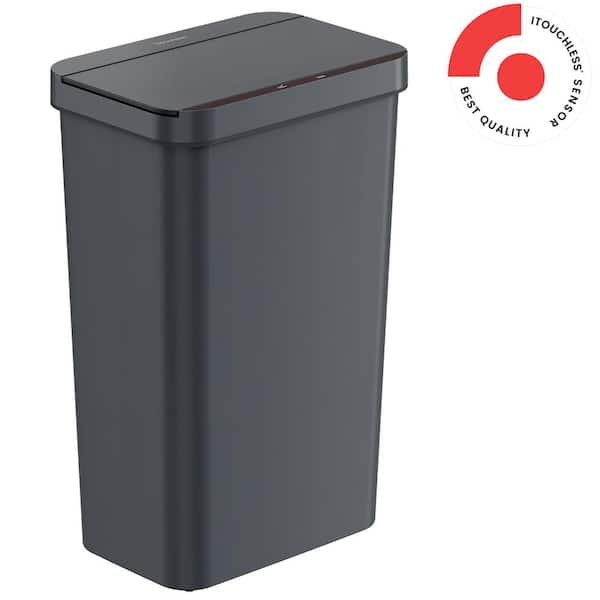The image displays a tall, modern gray or dark gray rectangular garbage can with a streamlined design and rounded corners. The lid features a ridge that likely serves as a hinge, allowing it to lift up smoothly. This sophisticated garbage can appears clean and stylish, lacking the traditional foot pedal for opening, suggesting it might have an automated function. On the upper right corner of the can, there is a red circular emblem with a red arc, accompanied by the text "iTouchless Sensor" and "Best Quality," forming a circular pattern around the emblem. This suggests that the garbage can operates with a touchless sensor, opening automatically when approached, combining functionality with a sleek, contemporary appearance.